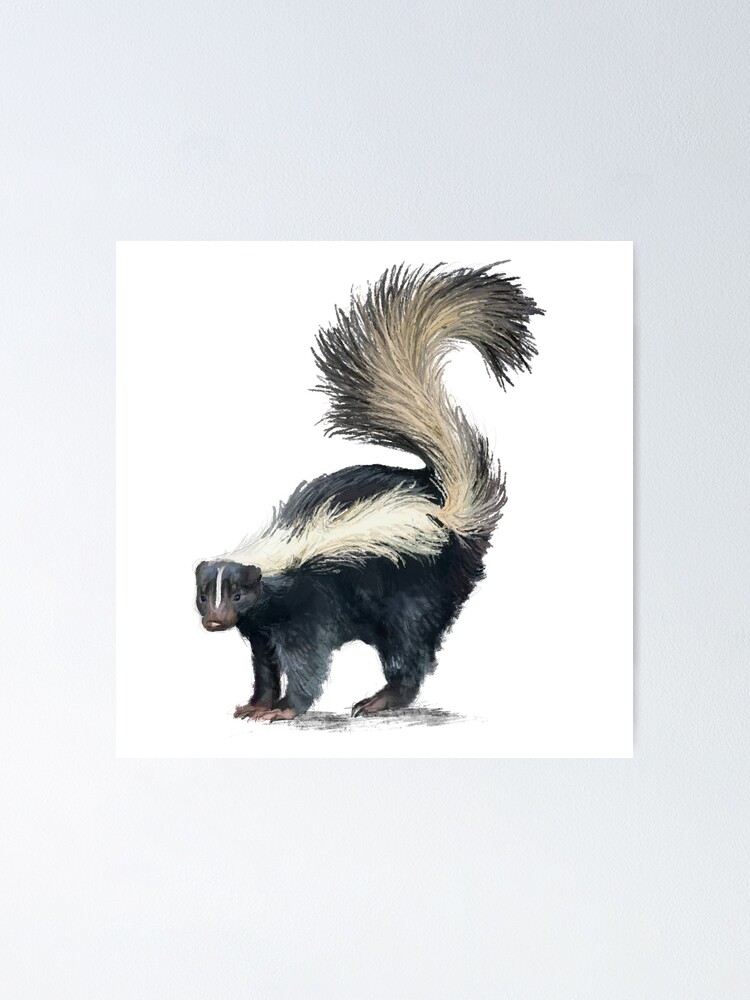The image is a digital mock-up of an art print featuring a detailed watercolor illustration of a skunk. The overall background is a light grey, with a square inset where the skunk print is displayed, and this square casts a shadow to the right side, creating a sense of depth. The skunk, predominantly black and white with hints of brown and reddish tones, is set against a plain white background. It is hunched slightly, suggesting it feels threatened and is ready to spray. All four paws are on the ground, though only three are visible due to the angle. Its tail is lifted and curled into an S shape. The skunk’s white stripe runs along its back and partially up the tail, blending the black and white fur to give a dark grey hue in some areas. Its face, turned slightly toward the viewer, features a white stripe, a small brownish nose, black eyes, and small ears. Beneath the skunk, a subtle shadow with a hint of ground texture is visible, enhancing the illustration’s dimensionality.